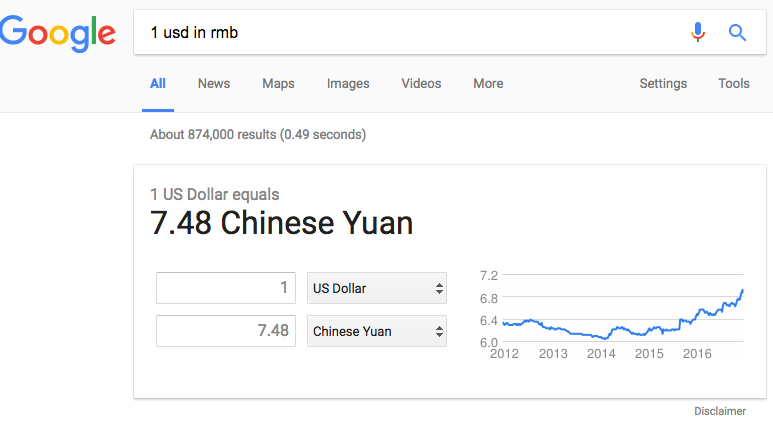This screenshot displays the results of a Google search query for the exchange rate between the United States Dollar (USD) and the Chinese Yuan (RMB). 

The interface is typical of a Google search results page. In the top left-hand corner, you can see the Google logo, composed of a capital blue "G," followed by lowercase letters: red "o," yellow "o," blue "g," green "l," and red "e." 

The search bar at the top of the page contains the query "one USD and RMB." To the right of the search bar, there is a small microphone icon for voice search, and a magnifying glass icon symbolizing the search function.

Beneath the search bar, there are several categories such as "All," "News," "Maps," "Images," "Videos," "More," "Settings," and "Tools." These options help to refine the search results. Below these categories, it indicates there are approximately 874,000 search results, retrieved in about 0.49 seconds.

The main content of the page prominently displays the current exchange rate: "1 US Dollar equals 7.48 Chinese Yuan." Beneath this, there is a graphical representation showing the historical exchange rate trends between the USD and RMB over a specified period.

The screenshot provides a comprehensive and detailed view of how one US dollar correlates to Chinese Yuan, along with additional features and functionalities typical of the Google search interface.